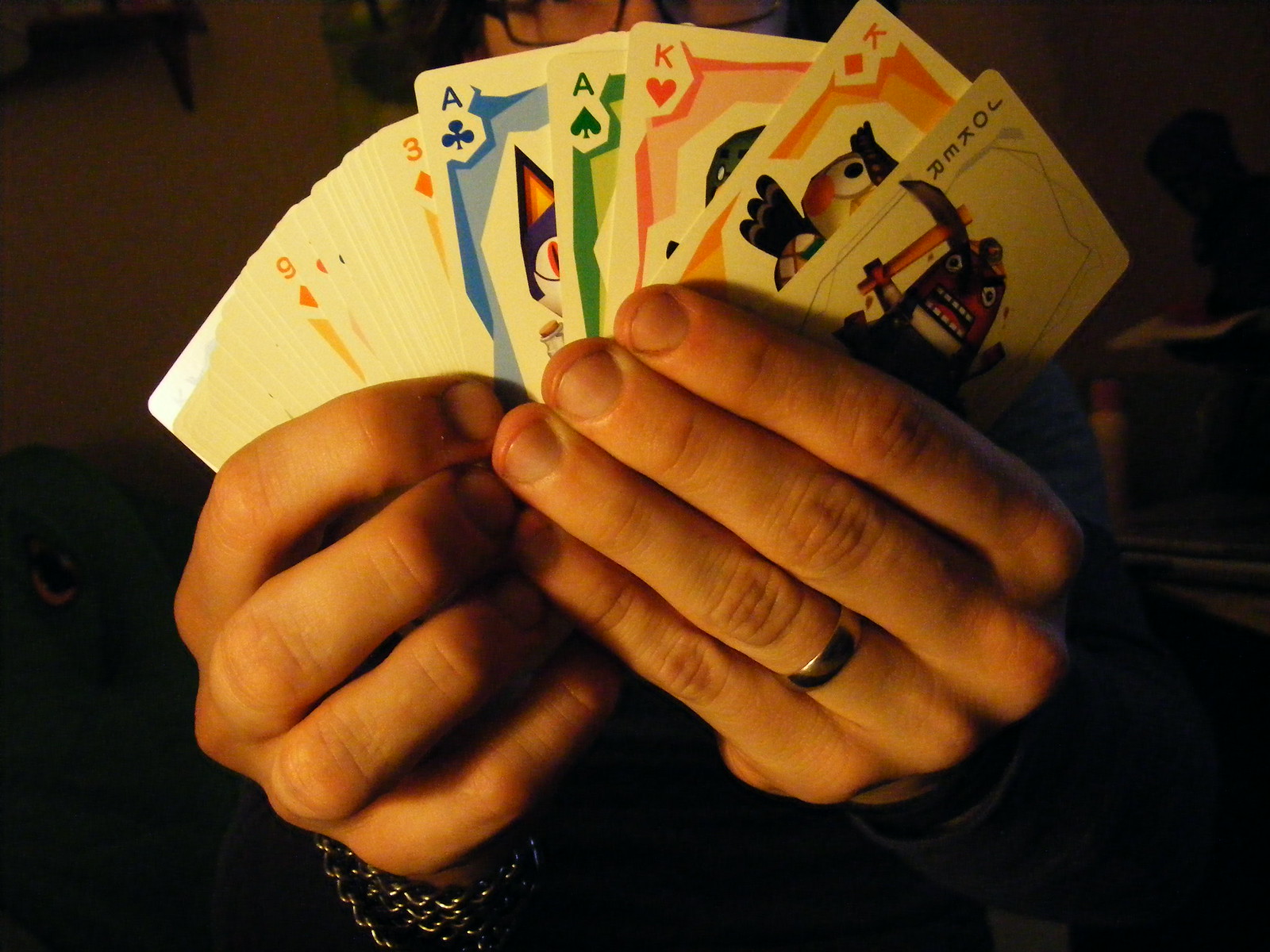In the image, a male figure is set against a dark background, holding a fanned-out deck of playing cards. The cards are spread in his hands, with the left-hand side of the deck more visible. Among the visible cards are the nine of diamonds, three of diamonds, ace of clubs, ace of spades, king of hearts, king of diamonds, and a joker. The playing cards feature a white background with cartoonish characters in place of the standard illustrations.

The man's left hand is partially visible, obscuring the nails, while the nails on his right hand are cut extremely short, down to the quick. He wears a wide wedding band made of either silver or white gold on his left hand. Additionally, he sports a silver chain bracelet on his left wrist. His attire includes a black shirt or sweater, discernible through its faint outline.